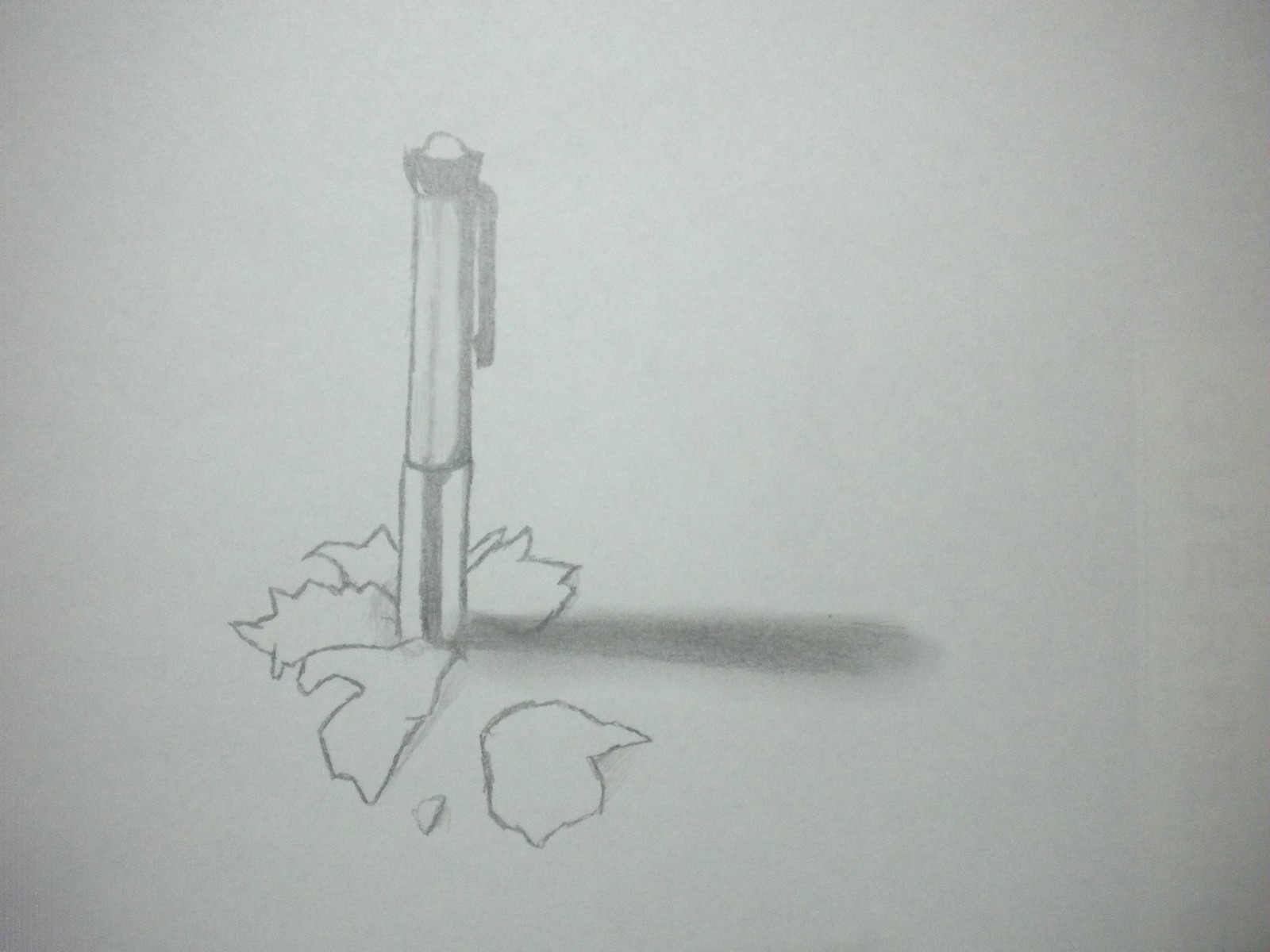A highly detailed pencil illustration depicts a pen, partially embedded into a surface up to about a quarter of its length. The pen features a classic clip, reminiscent of those once commonly used to secure pens in shirt pockets. Its retractable nib mechanism is visible at the top. Emerging from the embedded part of the pen are delicate, intricately drawn leaves, creating a striking contrast between the mechanical and natural elements. The artist has skillfully added the shadow of the pen, enhancing the realism of the image.